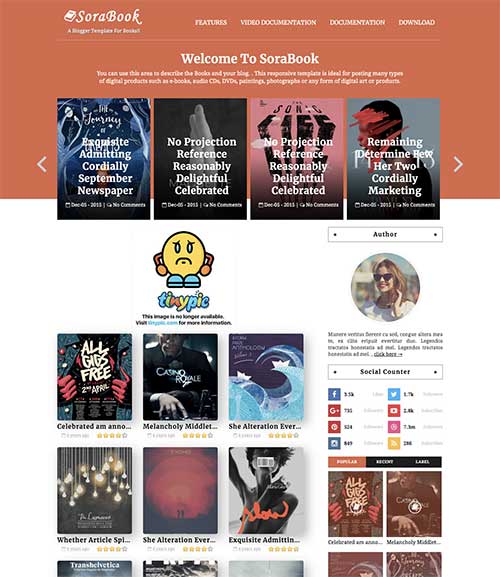This image is a screen capture of the Sora Book website, which appears to be a platform for purchasing books. Dominating the upper left corner is the Sora Book logo set against an orange bar. Directly below the bar, the text "Welcome to Sora Book" is prominently displayed. Beneath this welcoming message, there is a photo showcasing four featured books available on the site. Below these larger images, a series of smaller book thumbnails are visible, each accompanied by its title, though the text is too small to read clearly. To the right side of the screen, an informational bar provides details about the selected book. This bar includes subheadings such as the author and offers various social media integration options, including links to Facebook, Instagram, and Twitter.